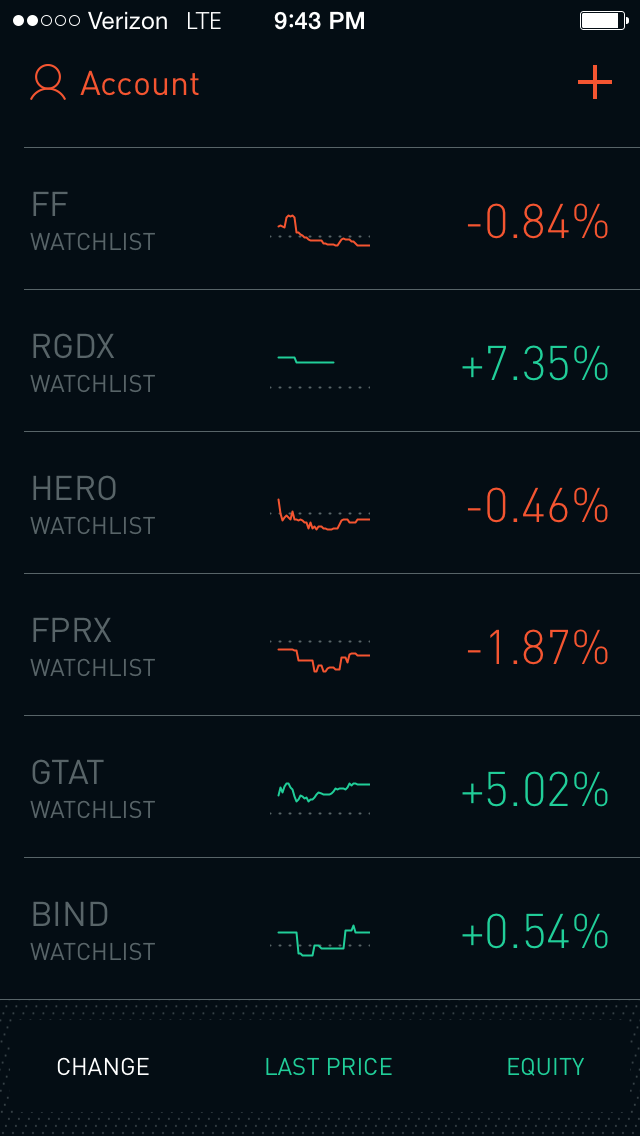**Detailed Image Description:**

This image is a cell phone screenshot depicting price changes of various financial instruments, displaying more height than width. The background of the screen is black. At the top, the status bar shows network information with "Verizon LTE" on the left, the current time "9:43 p.m." in the center, and a battery indicator on the right. Below the status bar, on the upper left-hand corner, there's a user account icon, while on the upper right-hand corner there's a plus sign, both in red font.

The main content is organized into several sections separated by thin horizontal lines. Each section details a different financial instrument, all formatted in a similar manner. The sections include:

1. **FF Watch List**: Displays a red graph indicating a percentage change of -0.84%.
2. **RGDX Watch List**: Shows a relatively flat green graph with a positive percentage change of 7.35%.

This pattern continues, presenting a total of six financial instruments, each identified by an alpha symbol, followed by the words "Watch List." In the center of each section, a graph is shown; it is red if the change is negative and green if positive. On the right side of each section, the respective percentage change is displayed, color-coded in red or green based on its value.

At the bottom of the screen, there are three distinct labels: "Change," "Last Price," and "Equity," listed from left to right. "Change" is written in white, while "Last Price" and "Equity" are colored green.